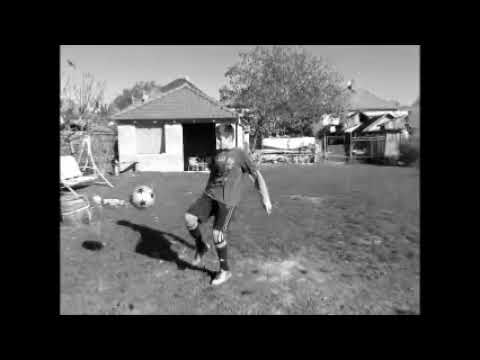In this black and white photograph framed by a large black border, a young boy, likely in his early teens, is frozen in action as he kicks a black and white soccer ball, which hovers in mid-air to the left side of the image. The boy is dressed casually in a t-shirt, black shorts, knee-high black socks, and light-colored shoes. His right arm is extended behind him, while his left arm is out of view. The striking contrast of light and shadow captures the silhouette of his form on the grassy field beneath him, complete with a few yellowed patches.

The scene unfolds in what appears to be a modest backyard likely situated in rural America. In the background stands a quaint house with an arched roof and a large open door, revealing a dark interior interrupted by the presence of a white chair at the bottom. To the left of the door, a closed window quietly punctuates the home’s facade. Beyond the central action, a tree towers over the right side of the yard, adding a natural frame to the composition. Adjacent to the tree sits another building, further enriching the backdrop with its subtle structure.

Completing this domestic tableau, the yard also features a swinging bench to the left, chairs scattered about, and a fence enclosing the grassy, yet slightly patchy, terrain under a hazy gray sky. The entire scene is imbued with a nostalgic touch, perhaps due to the visible low resolution reminiscent of a still frame from a bygone video.